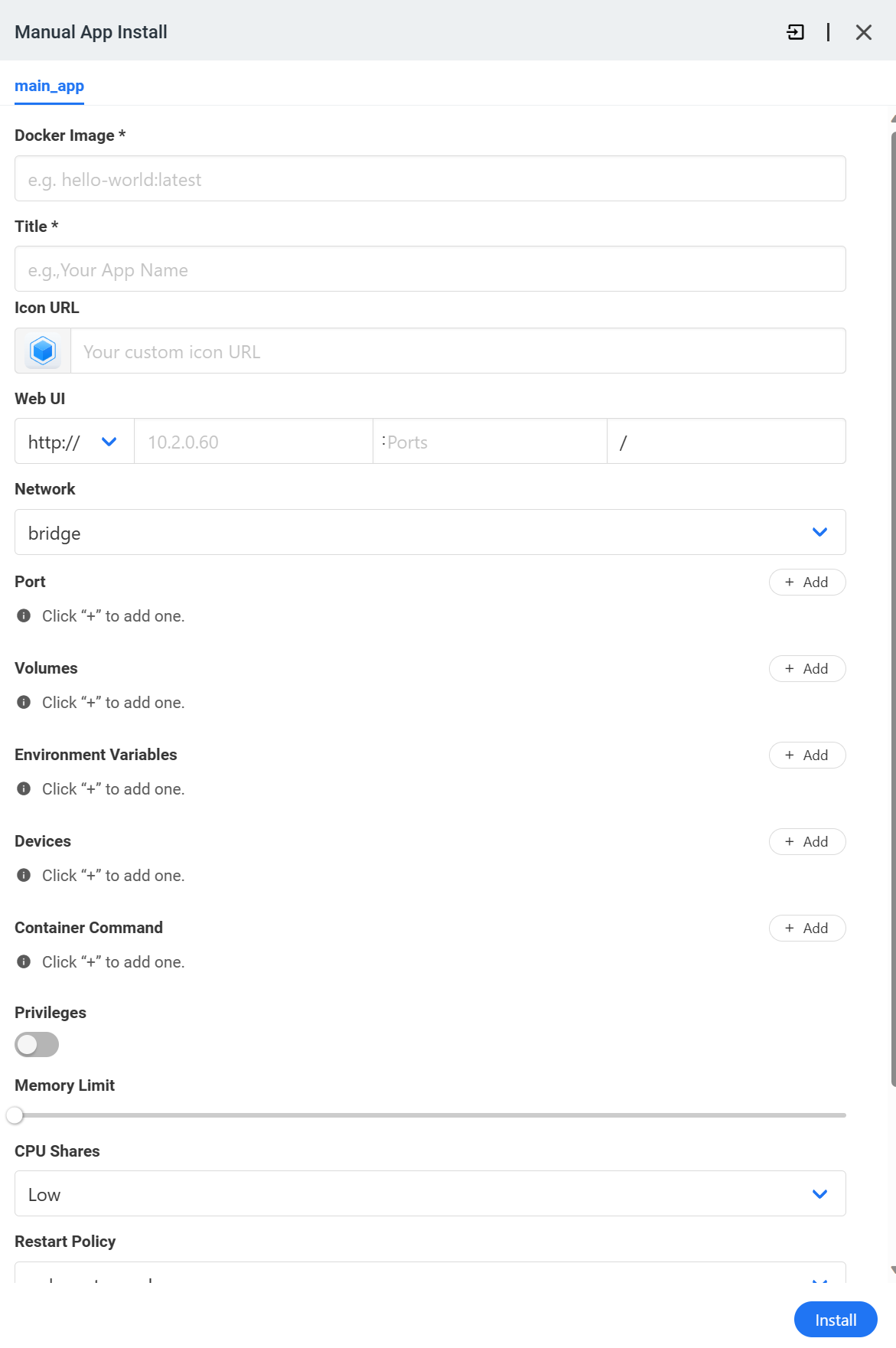This image is a detailed screenshot from a smartphone displaying a technical utility page for manual app installation. The header at the top of the screen is light gray with the text "Manual App Install" in a gray font. On the right side of the header, there are three gray icons: an 'X', a vertical line, and a square with a diagonal line through it.

Below the header, the background is white. The utility page is intended for users with technical skills. The first line of text, written in blue font, reads “main_app.” Below this line is a list of highly technical items:

- **Docker Image**: Users can input details related to a Docker image.
- **Title**: Field for entering the title of the app.
- **Icon**: Placeholder for adding an app icon.
- **URL**: Space provided to input the web URL for the app.
- **Web UI**: Customizations related to the web user interface.
- **Network**: Options for network settings, with "bridge" mentioned as a default option.

Further options prompt users to:
- Add a port by clicking the plus sign.
- Add volumes with a prompt, "Click + to add one," alongside a display of small boxes with plus signs and the word "Add."
- Add environmental variables in a similar manner.
- Add devices with the directive "Click + to add one."
- Add container commands via a plus sign icon.

Near the bottom of the screen, there is an option for setting privileges, indicated by a gray circle slider. Users can also set a memory limit with a gray line slider. Another setting, CPU shares, provides an adjustable option with a drop-down menu labeled "Low."

At the very bottom of the screen, there is a blue, rectangular button with rounded edges and white text that says "Install."